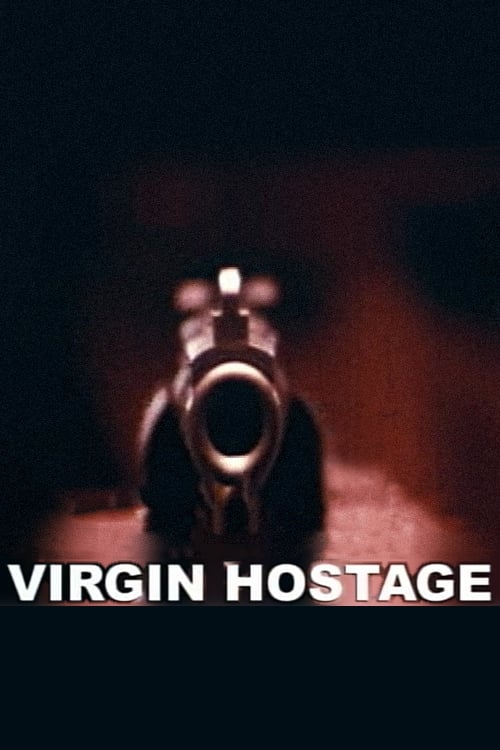The image is a dark, muted composition with a black background that slightly transitions to a dusty red hue. Dominating the center is a close-up of an old-fashioned gun, with its barrel pointed directly at the viewer, creating a stark and ominous focal point. The gun, which resembles a revolver with its round metal barrel, is highlighted by a selective light that accentuates the circular muzzle and the action piece used to cock it. Surrounding the sharply focused barrel, the rest of the gun fades into an unfocused blur, suggesting there might be a hand or a figure holding it. However, this detail, along with a man's face veiled in darkness, remains ambiguous due to the low light and blurred imagery. Below the gun, in bold white block letters, the phrase "Virgin Hostage" stands out above a solid black area that occupies the lower part of the image.